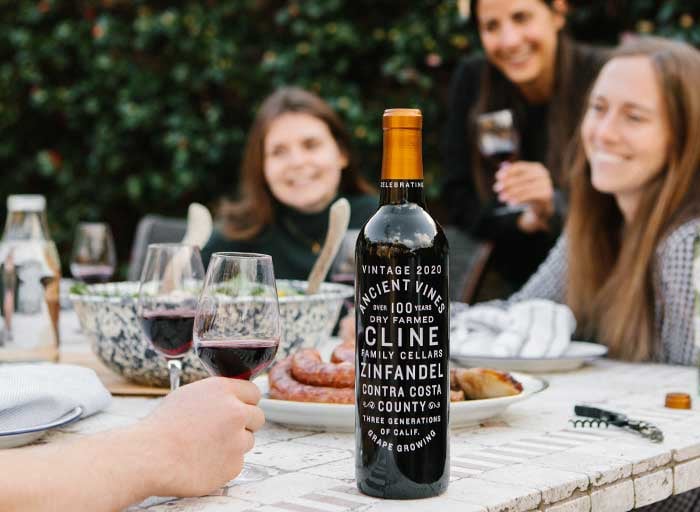This outdoor image captures a joyful gathering around a white marble table set against a backdrop of lush, green foliage. Dominating the foreground is a prominently displayed bottle of wine with intricate white text detailing, "Vintage 2020 Ancient Vines, Over 100 Years Dry Farmed, Klein Family Cellars, Zinfandel, Contra Costa County, Three Generations of California Grape Growing." Surrounding the table, we see three smiling women; two are seated, and one is standing in the middle, holding a glass of red wine. The table is adorned with a large salad bowl, plates, wine glasses, and a bottle opener. An anonymous hand, also holding a glass of wine, extends into the frame from the left. The stone table setting is complemented by white napkins and tablecloths, emphasizing the convivial atmosphere of friends enjoying fine wine and good food. The image, though slightly blurry in the background, clearly captures the expressions of the women and the rich details of the bottle's label, underlining the celebration of a cherished vintage.